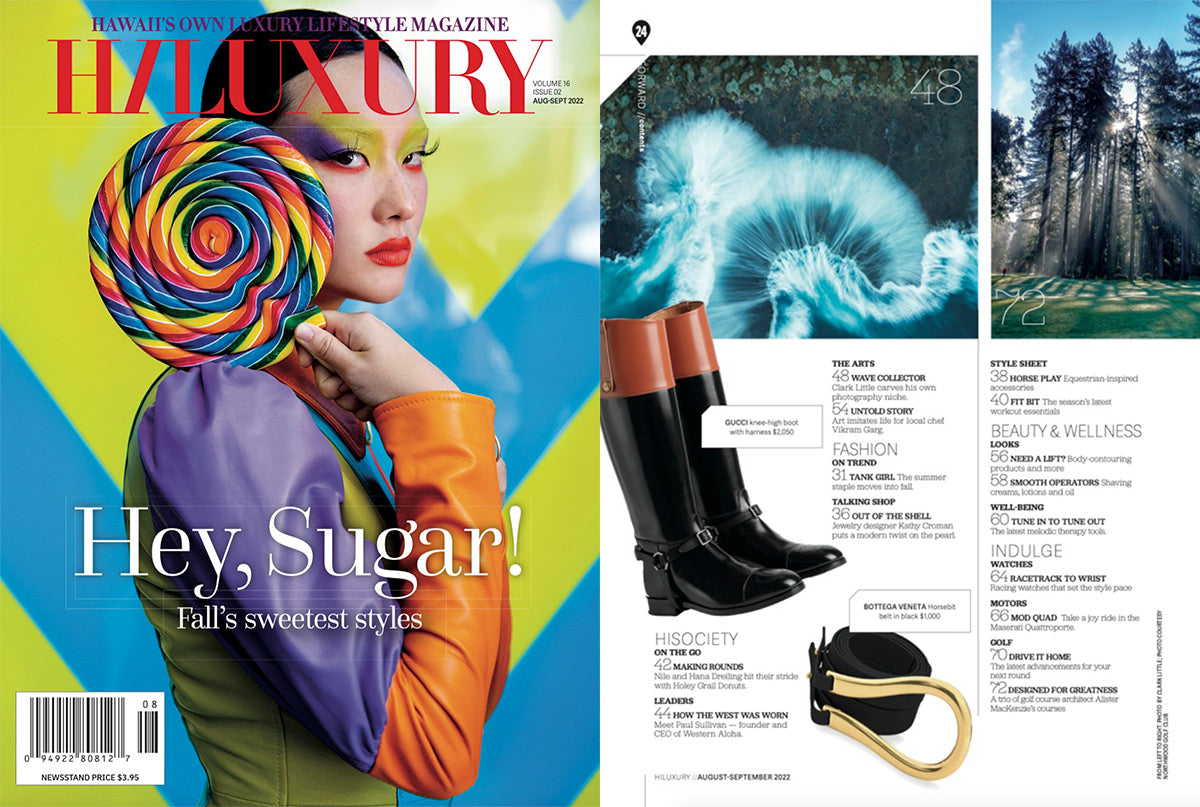The photograph is a rectangular composite image featuring both the front cover and index page of "High Luxury," Hawaii's own luxury lifestyle magazine, Volume 16, August to September 2022. Prominently displayed on the cover is a model, possibly of Pacific Islander descent, wearing a vibrant ensemble of a purple, orange, and yellow leather shirt with a triangular orange collar. Her striking makeup includes long false eyelashes, purple and lime green eyeshadow extending to her hairline, and vivid red lipstick. She is posing with a large, multicolored lollipop resting on her shoulder. The cover text includes the magazine's title "High Luxury" in red letters, along with captions such as "Hawaii's Own Luxury Lifestyle Magazine," "Hey Sugar," and "Fall's Sweetest Styles." A barcode is situated at the bottom left corner. Beside the cover, the index page is visible, detailing the magazine's contents under categories like arts, high society, indulge, beauty, and wellness, accompanied by small images depicting boots, trees, water, and a belt.